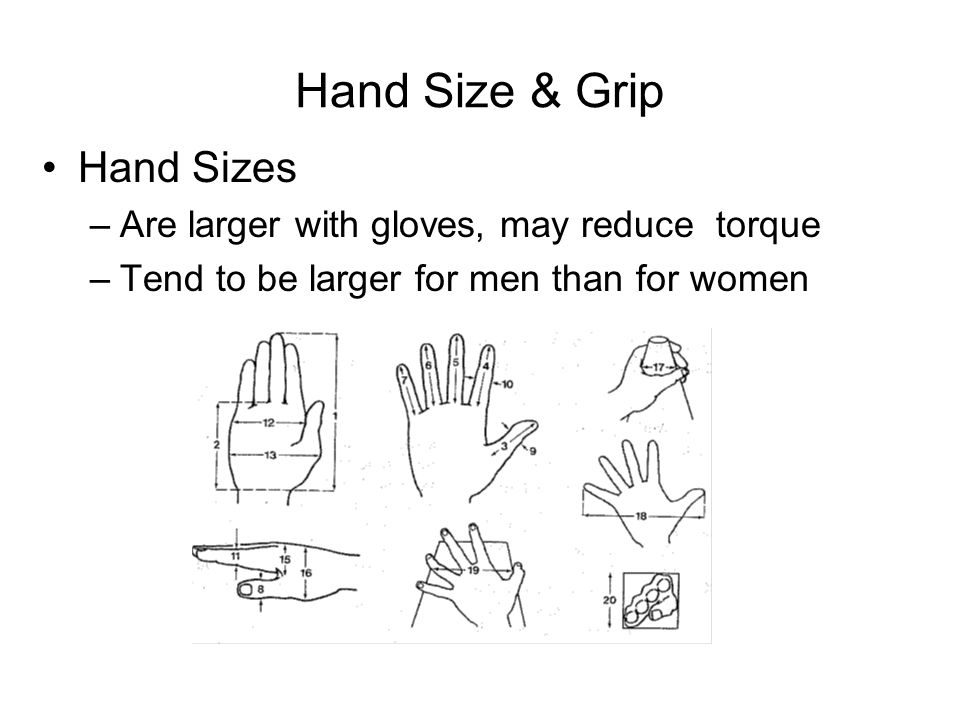This detailed black-and-white image illustrates the methodology for measuring hand sizes and grips, specifically for fitting gloves. At the top, the title "Hand Size and Grip" is prominently displayed in black lettering, with a black dot to the left and black hyphens introducing the subsequent points: "Hand sizes are larger with gloves, may reduce torque, tend to be larger for men than women." Below these statements, a series of six or seven detailed drawings show hands in various positions and perspectives, each surrounded by measurement lines and numbers (likely indicating units of measurement such as inches or centimeters).

The drawings include:
1. A palm-forward view, showcasing measurements from the middle of the palm to just below the fingers.
2. A palm-down view, detailing the lengths and distances between the fingers.
3. A side-on view with the thumb facing forward, displaying the hand’s dimensions.
4. A hand gripping a cone-shaped object.
5. A palm-spread view.
6. A hand gripping a square object.
7. A fist-like image highlighting the knuckles within a box.

Each hand drawing is meticulously labeled with measurement lines to help explain the sizes and dimensions, emphasizing the image’s instructional purpose.